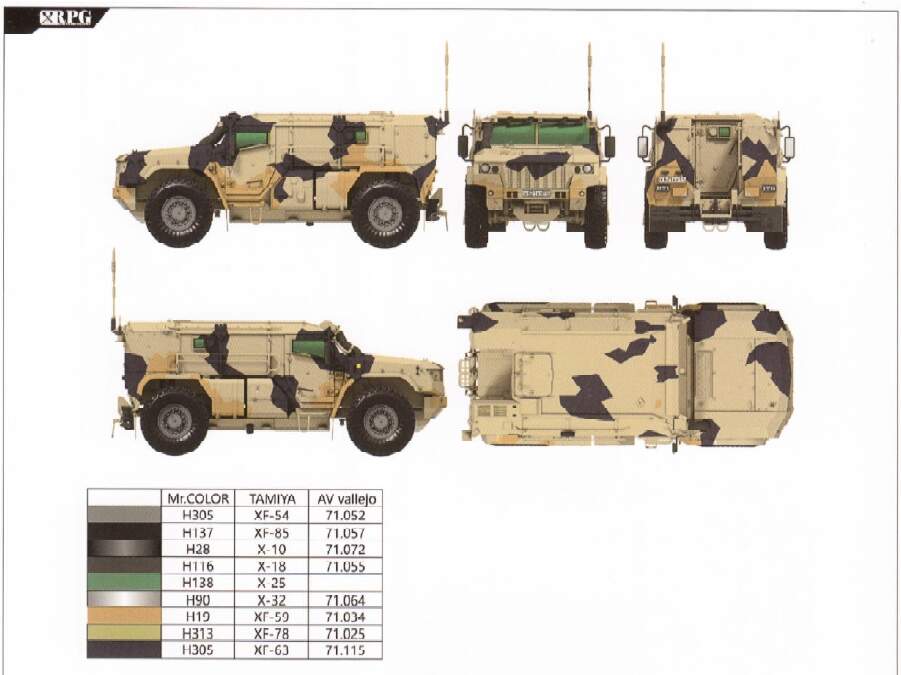The image showcases a comprehensive depiction of a military-style camouflage van from five different angles arranged in two rows. The top row presents the van's left side (showing its elongated, boxy body), front view (displaying distinctive green windows and a jeep-style grille), and rear view (highlighting an opening hatch and a small rear window). The bottom row features the right side and the top view of the van. The camouflage is predominantly a desert tan color with patches of dark gray and golden tan, and subtle green accents, creating an effective camouflage pattern suitable for desert environments.

In the lower left-hand corner of the image, there is a detailed color chart with four columns. The first column lists various colors including gray, black, green, silver, brown, and green, presumably the hues used in the camouflage. The subsequent columns are labeled "Mr. Color," "Tamiya," and "AB Vanager," each containing color model numbers corresponding to the different colors used in the van's design.